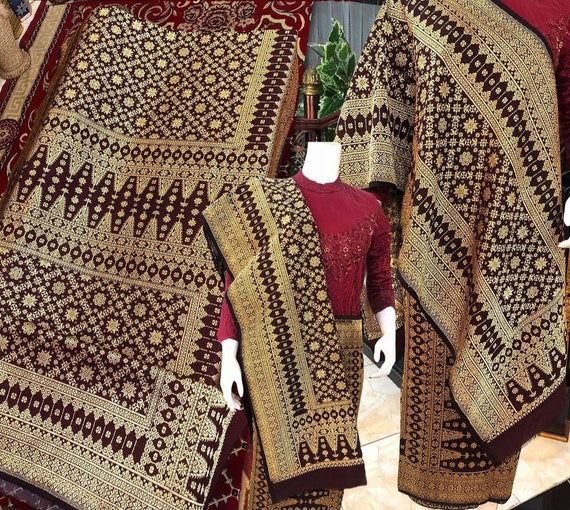The image features a detailed and richly textured scene centered around a white mannequin adorned in a maroon sweater with a V-shaped design across the chest and long sleeves. Draped over the mannequin's right shoulder and around its waist is a large shawl, or blanket, in earthy tones of brown and tan, intricately patterned with dark brown circles and a variety of shapes, including floral and coffin-like designs. This fabric, which exudes a traditional, possibly Middle Eastern or tribal aesthetic, is further highlighted by two zoomed-in shots placed on either side of the mannequin. The backdrop includes another mannequin also showcasing the shawl as a skirt, adding to the display of the textiles. The scene is complemented by additional elements such as a mahogany banister, a large green plant, and a hint of a rug, which together create a rich, immersive setting that amalgamates various cultural and vintage elements.